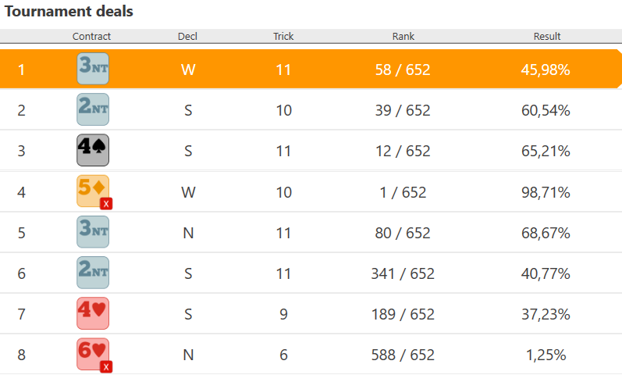This image is a screen capture, likely from a game interface focusing on tournament deals. The top of the image features a black header with the title "Tournament Deals" and is divided into five columns: Contract, DED, Trick, Rank, and Result. Each column is separated by a thin gray bar, and there are eight rows listed vertically.

**Detailed breakdown of the rows:**

1. **Row 1:**
   - **Contract:** Light blue box with "3NT" in blue font.
   - **DED:** White "W".
   - **Trick:** White "11".
   - **Rank:** 58 out of 652.
   - **Result:** 45.98%.

2. **Row 2:**
   - **Contract:** Blue-gray box with "2NT".
   - **DED:** S.
   - **Trick:** 10.
   - **Rank:** 39 out of 652.
   - **Result:** 60.54%.

3. **Row 3:**
   - **Contract:** Gray box with "4♠" (four of spades).
   - **DED:** S.
   - **Trick:** 11.
   - **Rank:** 12 out of 652.
   - **Result:** 65.21%.

4. **Row 4:**
   - **Contract:** Gold box with "5♦" (five of diamonds) and a red X.
   - **DED:** W.
   - **Trick:** 10.
   - **Rank:** 1 out of 652.
   - **Result:** 98.71%.

5. **Row 5:**
   - **Contract:** Blue-gray box with "3NT".
   - **DED:** N.
   - **Trick:** 11.
   - **Rank:** 80 out of 652.
   - **Result:** 68.67%.

6. **Row 6:**
   - **Contract:** Blue-gray box with "2NT".
   - **DED:** S.
   - **Trick:** 11.
   - **Rank:** 341 out of 652.
   - **Result:** 40.77%.

7. **Row 7:**
   - **Contract:** Pinkish-red box with "4♥" (four of hearts).
   - **DED:** S.
   - **Trick:** 9.
   - **Rank:** 189 out of 652.
   - **Result:** 37.23%.

8. **Row 8:**
   - **Contract:** Red-pink box with "6♥" (six of hearts).
   - **DED:** N.
   - **Trick:** 6.
   - **Rank:** 588 out of 652.
   - **Result:** 1.25%.

Each row provides a detailed summary of a contract deal, including the number of tricks taken, the rank among participants, and the resultant percentage score.